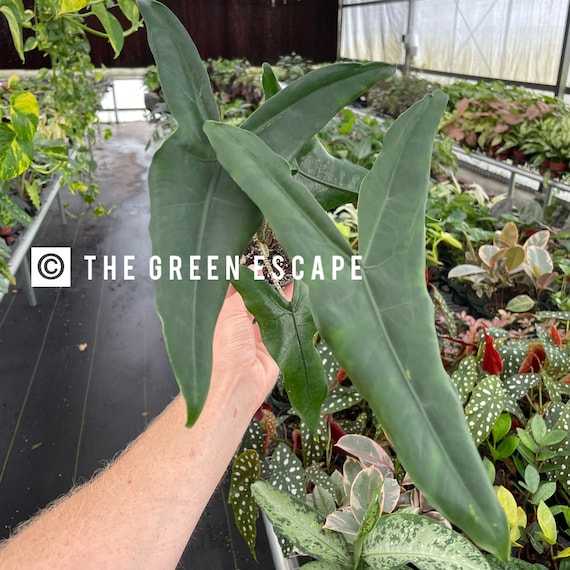The photograph captures an indoor garden area, seemingly a greenhouse or plant nursery. The setting is filled with a variety of plants, arranged neatly in rows on tables that span the area. The plants display a diverse array of foliage, with leaves ranging in color from vibrant green to shades of yellow and red, and varying significantly in size and shape. 

In the foreground, a white hand emerges from the lower left corner, grasping a plant with distinctively shaped leaves. The leaves are elongated, thin, and pointy, resembling arrowheads with a unique structure—each featuring a single point at the bottom and two points forming a V at the top. These leaves are nearly the length of the person's forearm, accentuating their unusual appearance.

The ground of the building is a dark gray, while the background includes contrasting black and white sheets. Prominently displayed in the center of the image is the text "The Green Escape" written in white, accompanied by a logo on the left and a copyright symbol on the right. The overall ambiance suggests an exotic collection of plants not commonly seen outside specialized environments such as nurseries or greenhouses.